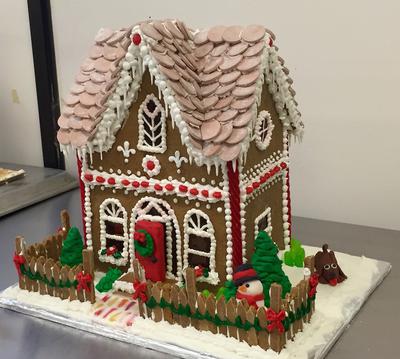This detailed picture depicts a traditional Christmastime gingerbread house set inside on a grayish-colored table. The house, perched on a small raised platform, is a charming two-story gingerbread structure adorned with a plethora of frosty decorations. The brown gingerbread house features windows outlined in white icing and a front door painted red with a green wreath, evoking a cozy winter look. The roof, intricately designed with what appears to be candy wafers and decorated with small circular candies to mimic shingles, adds a delightful touch. Surrounding the house is a quaint brown fence garnished with pine boughs, enclosing a winter wonderland scene with green pine trees and a jolly little snowman. The snowy effect is masterfully created using white frosting, which also outlines the entire house. Additionally, a small dog adds a touch of whimsy to the festive display. Overall, the craftsmanship of this gingerbread house is exceptional, embodying both traditional and meticulous holiday spirit.